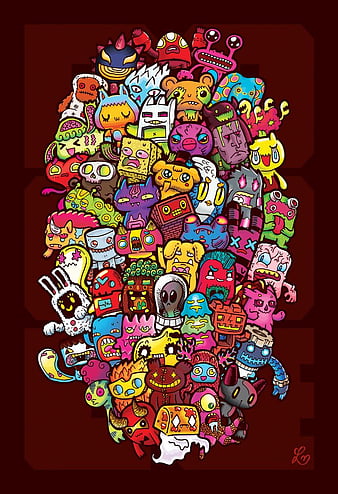The image is a digital wall art in portrait orientation, featuring a dense and colorful cluster of hand-drawn cartoon characters set against a deep eggplant-purple background with a dark brown border. The characters, approximately fifty in total, are intricately stacked on top of each other with no space in between, creating a vibrant and chaotic scene. They represent a wide variety of forms including rabbits, marshmallows, bears, scary creatures, birds, Spongebob-like figures, monkeys, aliens, robots, and crabs. This collage of characters showcases an extensive palette, displaying greens, yellows, oranges, reds, blues, pinks, purples, and many other colors from across the spectrum. In the bottom right corner of the artwork is a simple, light orange signature resembling the letter 'L', adding a personal touch from the artist.